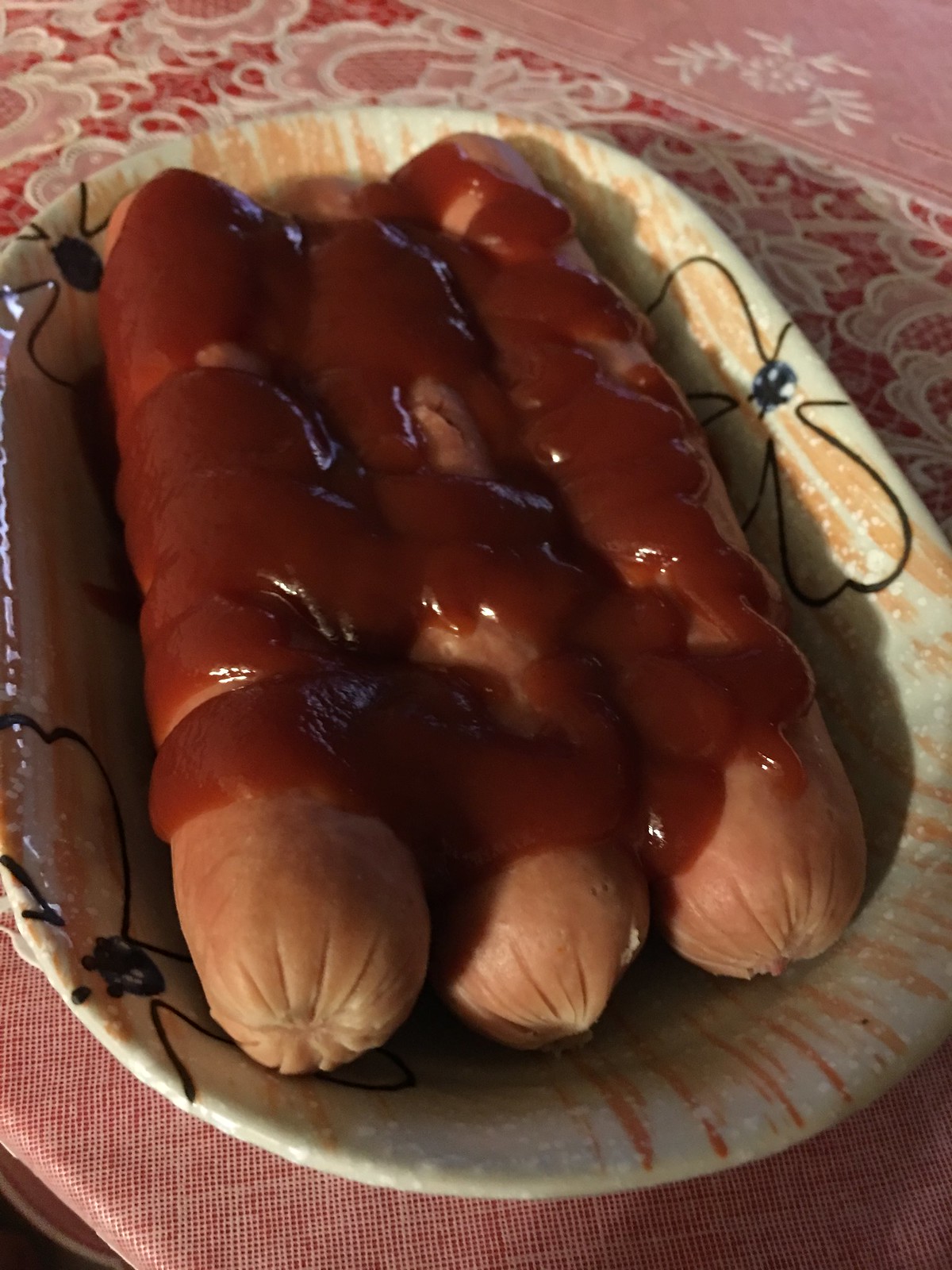The photograph features a close-up of a decorative platter set atop a vintage floral tablecloth. The platter itself is white with a subtle yellowish hue, accented by an orange-coral design and outlined black floral sketches. This elegant, yet slightly retro design is accentuated by green stripes that run across the platter. 

Three hot dogs, generously covered in a darker shade of red ketchup, sit in the center of the platter, so much so that they are nearly obscured by the condiments. The image is taken from a 45-degree angle, providing a slightly elevated yet angled perspective of the scene.

The tablecloth beneath features a nostalgic, grandmotherly design with intricate doily-like floral patterns in red, white, pink, and touches of yellow. The pattern appears textured, almost 3D, giving the tablecloth a vivid, tactile quality. This detailed setup combines to create a charming and vibrant composition.